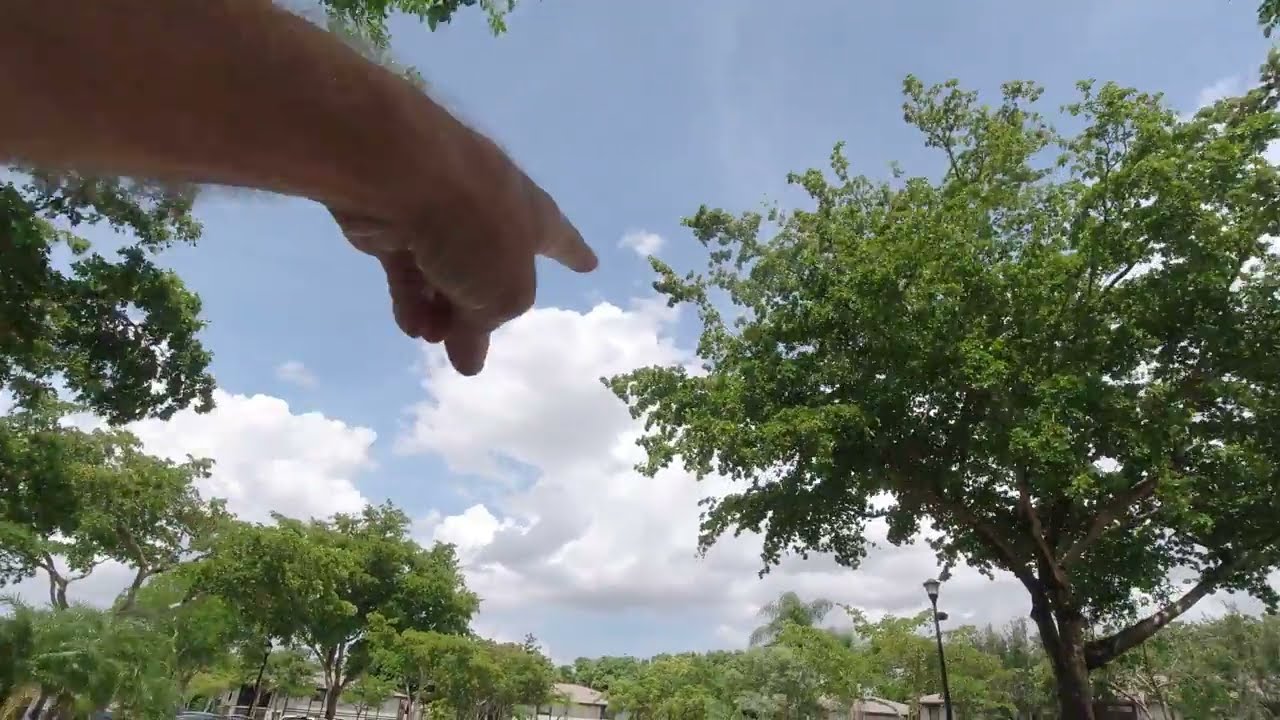The photograph captures a serene outdoor scene dominated by a light blue sky scattered with large, white fluffy clouds near the horizon. Emerging from the top left corner, a person's hairy, white forearm extends into the frame, with their index finger pointing upwards towards a large, leafy tree that occupies much of the right-hand side. This prominent tree, possibly an oak, is surrounded by an assortment of other green shade trees, indicating the growing season of late spring or summer. The landscape also features several white buildings with tan or grayish roofs, partially obscured by the verdant foliage. A classic black streetlamp stands to the immediate left of the tall tree, adding a touch of urban charm to the otherwise natural setting. In the distance, more treetops and the tops of additional buildings are visible, blending harmoniously into the lush, green environment.